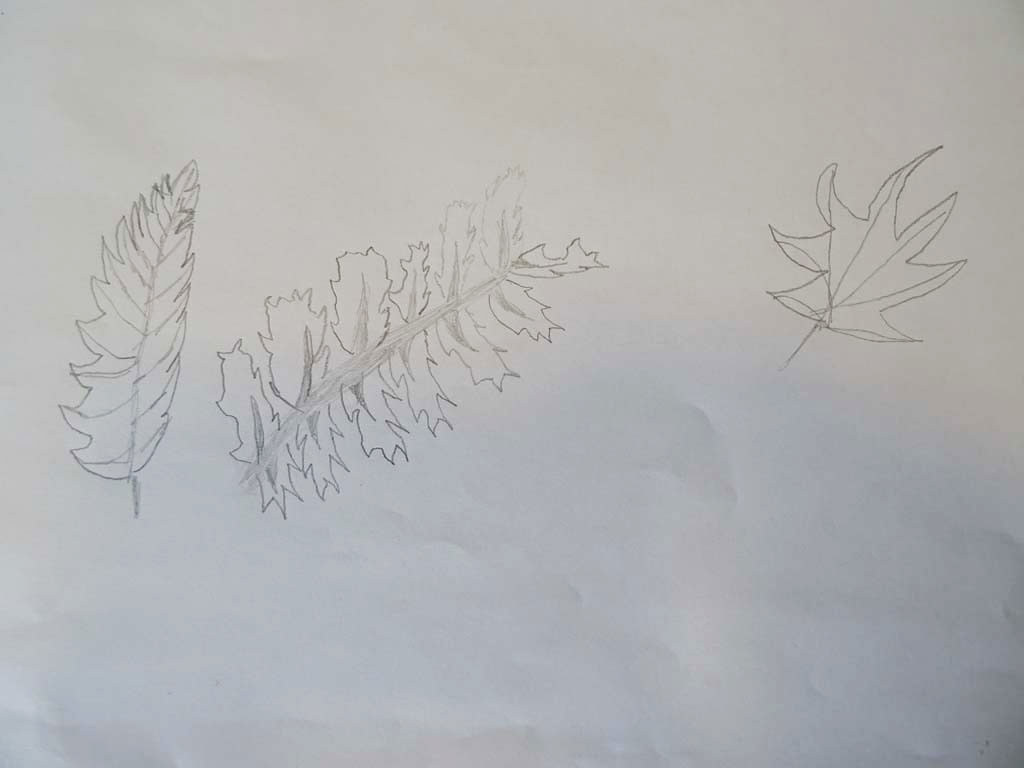A pencil drawing on a crumpled, white office copy paper features a variety of leaves, showcasing attempts at different styles and detailing techniques. The paper has noticeable creases and wrinkles, suggesting it has been handled roughly. On the right-hand side, there's a simple, seven-pointed leaf with basic line details, lacking significant refinement. The left-hand side displays a more intricate leaf resembling a feather, with serrated edges and a central vein. In the middle, a long stick runs horizontally with six smaller lines extending from it, each bearing a finely detailed serrated leaf on both sides. The overall sketch appears to be a practice exercise in capturing different leaf textures, edges, and shading with a pencil.